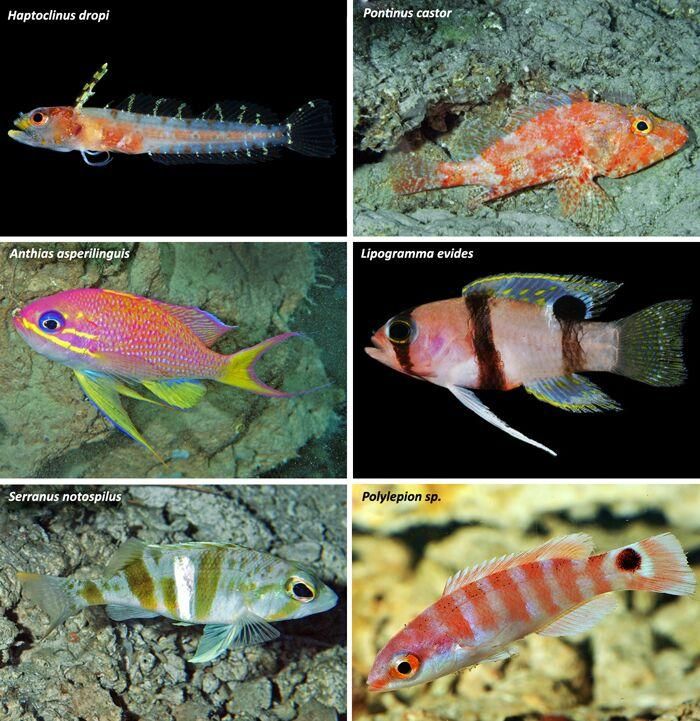This image collage presents six vibrant photographs of different exotic, deep-water fish species, arranged in three rows with two images each. The fish are displayed against varied backgrounds, with some set against stark black backdrops typical of deep-sea photography. 

1. **Haptoclinus dropi** (Top Left): This translucent, elongated fish features delicate tendrils sprouting from its back and belly, with a blend of blue, red, and yellow coloring. Its nearly see-through fins add to its ethereal appearance.

2. **Pontinus castor** (Top Right): Resembling a cross between a red snapper and a lionfish, this reddish-white fish rests on rocky terrain. Its scales exhibit orangish and white hues, lying at the rock bottom with distinctive features.

3. **Antheus asperilingus** (Middle Left): This tropical fish showcases a bright pink body adorned with neon yellow fins and prominent yellow stripes. Its face is marked with these stripes, and it has striking blue eyes, contributing to its vivid appearance. Rocks are visible in the background.

4. **Lipogramma evides** (Middle Right): Against a black background, this pink fish is characterized by three vertical black stripes — one around its eye, one on its midsection, and one near its tail. Its fins are highlighted with blue and yellow accents.

5. **Serranus notospilus** (Bottom Left): Featuring a gray body with green stripes and yellow accents, this fish is seen swimming above a rocky sea floor. 

6. **Polylepion sp.** (Bottom Right): This small, slender, white fish is detailed with orange stripes and an orange stripe across its eye. It also features a distinctive red circular dot on its tail fin, providing a striking contrasting pattern.

Each fish is captured with its scientific name embossed in white or black text, ensuring clear identification of these mesmerizing deep-sea inhabitants.